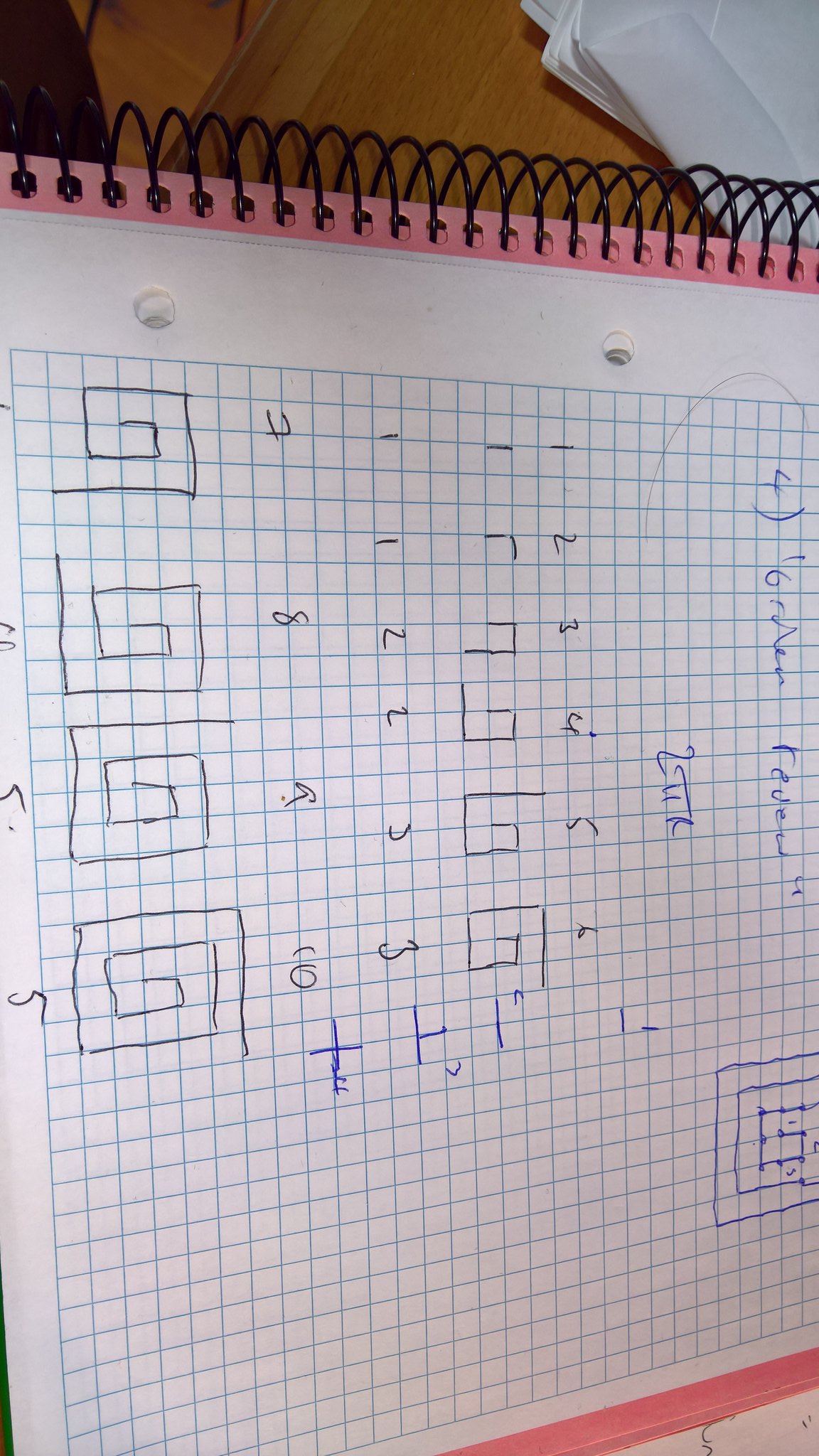The image showcases a meticulously organized graph on a binder full of paper. At the top, the metal wire of the spiral plastic binder is visible, securing the sheets together. The edge of the paper features a distinct pink line at the top, followed by a blank white space. Just below this space, there are a series of holes punched into the paper. 

The centerpiece of the page is a graph comprising blue-lined squares, extensively annotated with various writings. On the left side of the graph, annotations start from the left, move right, ascend slightly, return leftwards, descend again, and then curve back towards the right in a swirling pattern. 

Beneath this main graph, there appears to be another, nearly identical image, distinguished by an upward line on the left side. This line extends towards the right in a meandering fashion. Further down, a third similar image features another line that arcs over the top towards the right and then descends again.

At the bottom of the graph on the left side, several annotations are visible, including the number 5. Above this section, there are numerals such as 4, 8, 7, and 10 scattered across the page. Many more designs, seemingly similar in nature, are also present.

The annotations are predominantly in black ink, complemented by lighter blue ink drawings. At the bottom, there are some crossed-out sections, and in the bottom right corner, a square design filled with blue dots can be seen. Above this design, a section of cursive writing is present, adding a final touch of detail to the image.